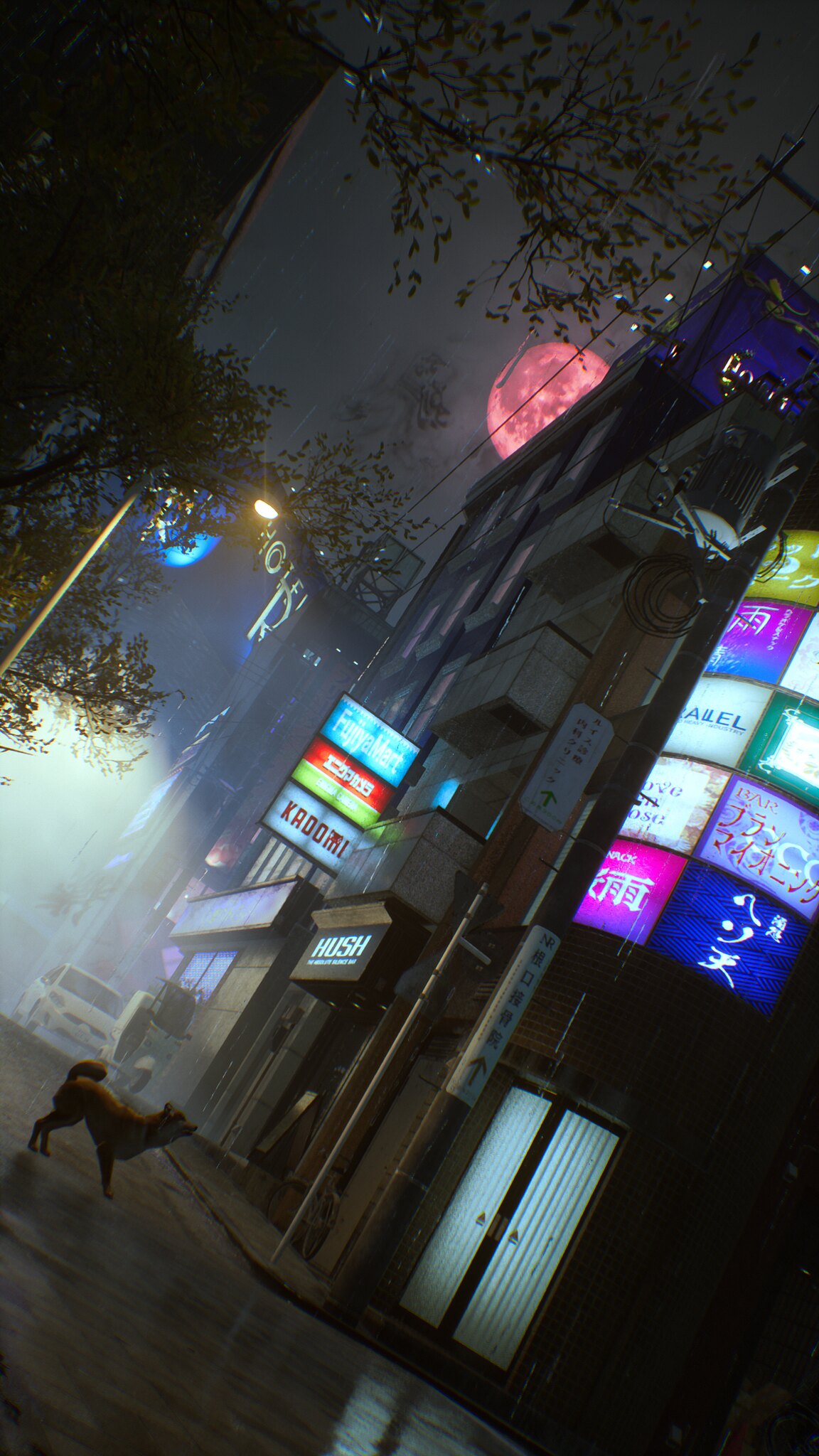This image captures a nighttime urban scene with an angled perspective, adding a dynamic, slightly sideways view. The setting features the side of a multi-story building, likely around four stories tall, adorned with various illuminated signs, many of which appear to be in an oriental script, suggesting an international location. The building dominates the right side of the image, extending from the bottom right corner almost to the top, and then horizontally toward the center. There are several billboards lit up along its side, offering a contrast to the dark night sky.

In the foreground, a large, fluffy brown dog stands on a concrete area near the base of the building, facing to the right and seemingly fixated on the structure. The concrete stretches upwards and to the left, and above it, trees with leaves outlined against the dark sky intrude into the upper left of the image. A streetlight on the left side casts a subtle glow.

Further back, a small white car is parked on a side road. Toward the top left, a red-tinted moon is partially visible above the building, adding an eerie, unique touch to the scene. The composition of the photo, combined with the distinct lighting and elements like the moon and signs, creates a vivid, almost cinematic moment in time.